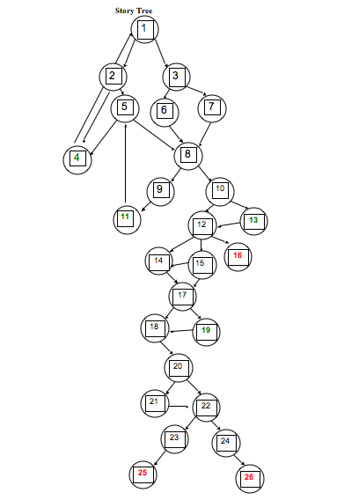The image depicts an intricate diagram titled "Story Tree" at the top. The diagram begins with the number "1" enclosed within a rectangular or square box, which is further surrounded by a circle. From this central shape, arrows branch out in various directions, connecting to numbers "2" and "3" on opposite sides. These numbers are also enclosed within squares or rectangles, each surrounded by circles. This pattern progresses with arrows extending from each numbered circle to new numbers, continuing until the highest number, "26."

The majority of the numbers are written in black text, though some are colored differently for emphasis or categorization. Specifically, numbers "4", "13", "19", and possibly "11" appear in green text, though distinguishing between black and green text is challenging. Numbers "16", "25", and "26" are notably in red text, indicating they may hold particular significance. Overall, the diagram presents a complex network of interconnected nodes, suggesting a branching narrative or decision tree structure.